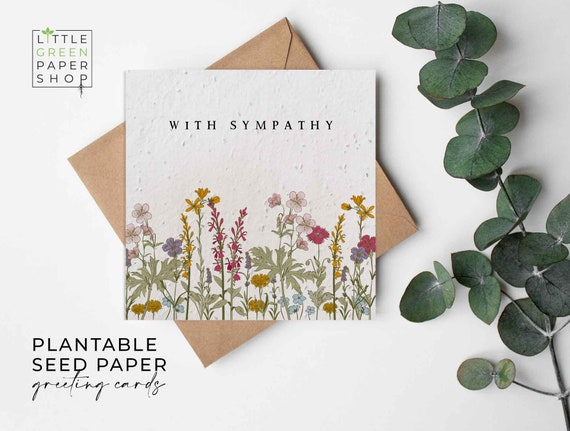The image features a square white card with black lettering in the middle that reads "With Sympathy." Below this text, there are illustrations of various flowers in yellow, purple, and pink hues. The card's background has a textured surface with small black dots. In the top left corner of the card, a small square prominently displays "Little Green Paper Shop" with "Green" written in green and the rest in black; the dot on the "i" in "Little" is shaped like a green leaf. The bottom left corner reads "Plantable Seed Paper," followed by "Greeting Cards" in cursive. This card is placed on top of a brown envelope, which is tilted so that its corners are visible. To the far right, a branch with dark, thick green leaves casts a light gray shadow on the white surface underneath. The image is set against a white background, creating a clean and crisp appearance.